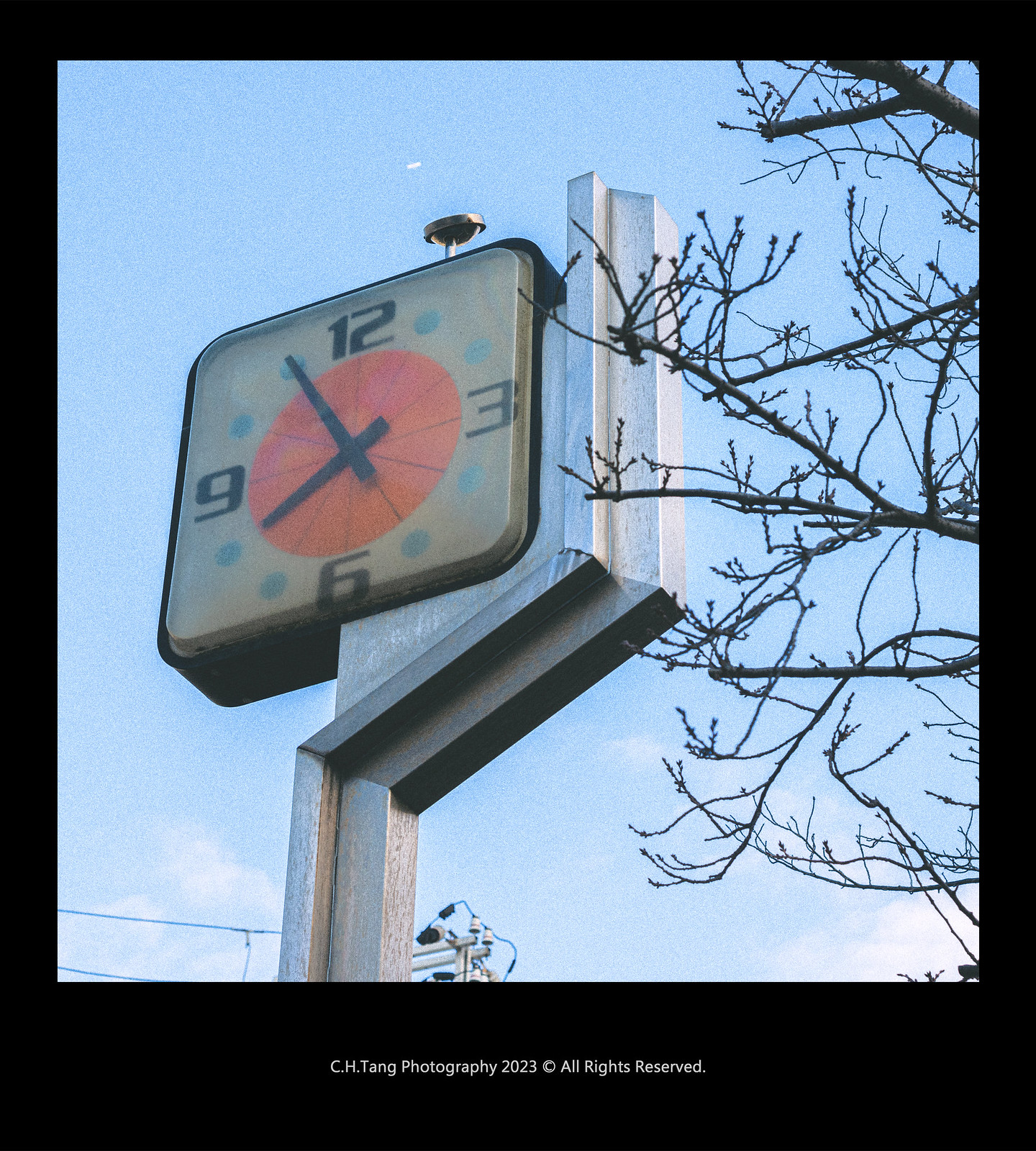This detailed photograph captures a large, square, retro-style outdoor clock mounted on a unique, silvery chrome, zigzag metallic structure. The clock itself is bordered in black, with a predominantly white face featuring light blue dots representing the numbers 1, 2, 4, 5, 7, 8, 10, and 11. Bold black numerals mark 12, 3, 6, and 9, emphasizing a vintage aesthetic further highlighted by a pastel orange circle at the clock's center. The black hour and minute hands show the time as 7:55. At the top of the clock is a small metal protuberance, adding to its intricate design. The photograph includes a glimpse of the natural environment, featuring the upper half of a tree trunk with bare branches on the right and a clear blue sky with a few wispy white clouds. Additionally, a part of a power line is visible in the lower left corner. The image is framed in black, with the bottom center of the border adorned with white lettering that reads, "C.H. Tang Photography, 2023 ©, all rights reserved."